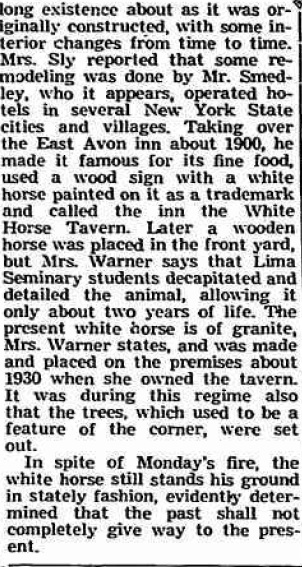The image is a clipping of a newspaper article with a white background and black text, starting mid-sentence, detailing the history of the White Horse Tavern. It reads: "Long existence about, as it was originally constructed with some interior changes from time to time. Mrs. Sly reported that some remodeling was done by Mr. Smedley, who operated hotels in several New York State cities and villages. Taking over the East Avon Inn around 1900, he made it famous for its fine food and used a wooden sign with a white horse painted on it as a trademark, renaming the inn the White Horse Tavern. Later, a wooden horse was placed in the front yard, but Mrs. Warner noted that Lima Seminary students decapitated and vandalized the figure, giving it a lifespan of only about two years. The current White Horse, made of granite, was placed on the premise around 1930 when Mrs. Warner owned the tavern. This transformation included the introduction of trees, a noted feature of the area. Despite a recent fire on Monday, the granite White Horse still stands tall, symbolizing the resilience of the past amid present challenges."